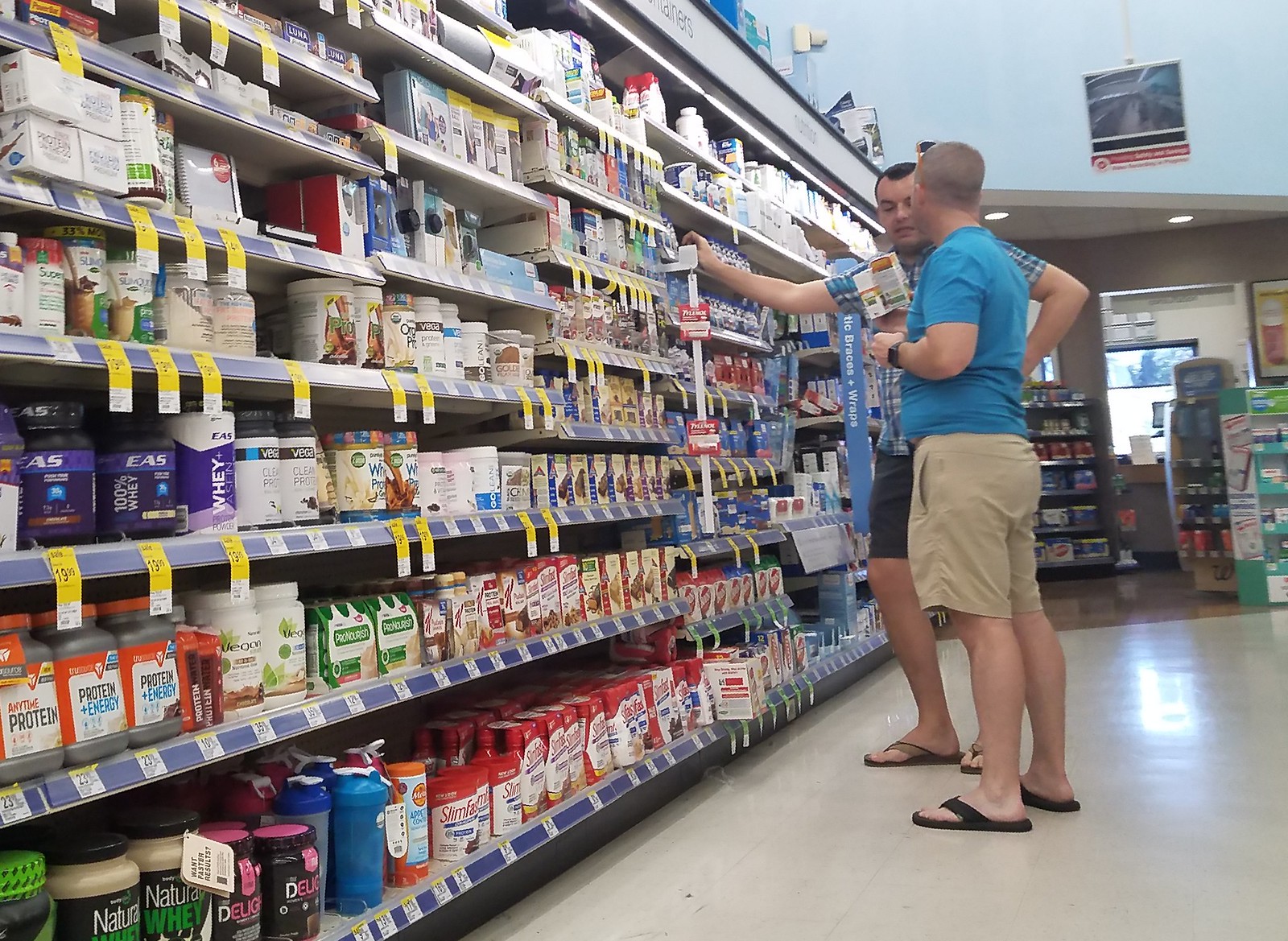In this grocery store aisle, two men engage in conversation face-to-face. The man in the foreground has his back to the camera, dressed in a blue short-sleeved shirt, khaki shorts, and slippers. Opposite him, the second man wears a short-sleeved flannel shirt paired with black shorts and slippers. The aisle is lined with various protein products and other boxed and containerized food items. These protein products are predominantly displayed on the right side of the image. Bright yellow tags dangle from the shelves, highlighting special offers or prices for the items.